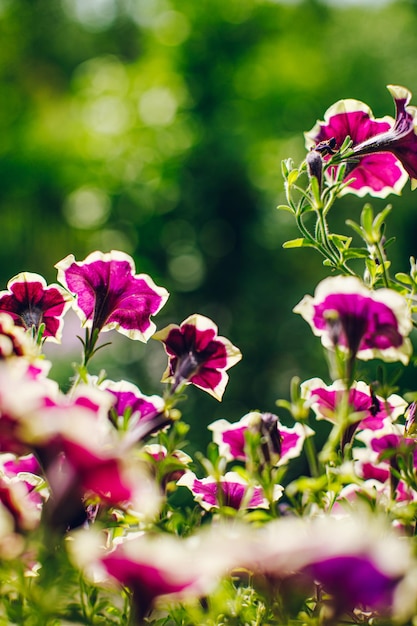This detailed close-up photograph captures a sunny day in a meadow, focusing on around 10 to 15 small petunia flowers. The image is taken from a ground perspective, with a blurry green background hinting at surrounding vegetation. The flowers, of varying sizes and in different stages of bloom and decay, predominantly exhibit a deep purplish-red hue with distinctive white edging around their round petals. Most of the flowers are facing away from the camera, making it difficult to see their centers clearly. Despite the lack of sharp focus on the closest flowers, the natural sunlight enhances the vibrant colors of the petunias, highlighting their beauty amidst some visible blades of grass at the bottom of the image.